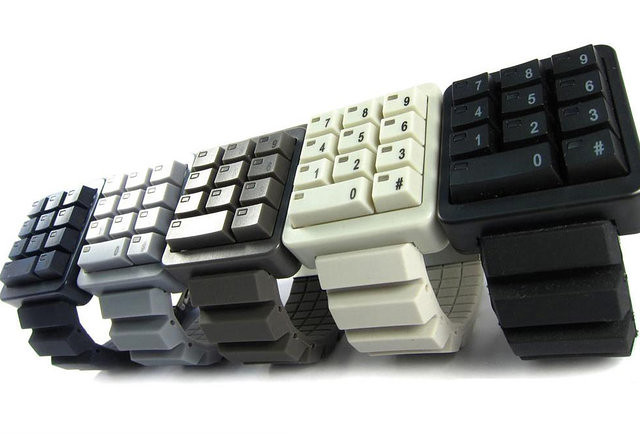This photograph showcases a close-up view of five wristwatch-like devices lined up side by side against a featureless white background. Each device features a square face resembling a numeric keypad with buttons labeled 0-9 and a pound sign (“#”). The wristbands, which appear to be made of flexible materials, are designed with multiple rectangular segments that allow them to expand. The colors of the devices from left to right are dark blue, light gray, brown, white, and black. Notably, the two devices on the right have clearly marked numeric keys, while the remaining three simply display small square emblems where numbers would typically be. These unique gadgets could potentially serve as wireless numeric keypads for conventional keyboards or might be attachments for mobile devices, offering a tactile interface for dialing numbers.